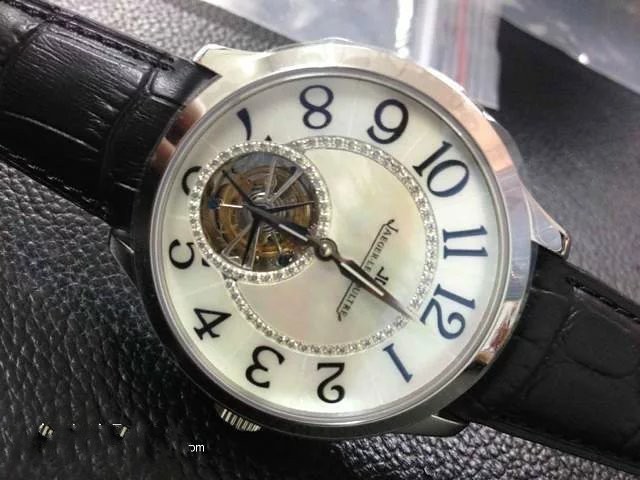This is an intricate close-up color photograph of a high-end luxury watch, possibly a Jaeger LeCoultre. The watch face, rotated to the right so that the 12 is at the 3 o'clock position, showcases the time set precisely at 6 o'clock. The face is an exquisite off-white, pearl-like color, accented by a small circle around the center, encrusted with fake diamonds, and surrounded by a silver band. The brand name, partially visible and hinted as "Jaeger LeCoultre," is delicately written in black. Prominently featured are black hour and minute hands with white stripes.

The watch has a distinctive small open area at the lower part, covering the numbers 5 through 7, revealing the intricate gears and inner workings of the clock. This open section is outlined with a circle of small fake diamonds, adding to the luxurious feel.

The watch band is a striking black, with a pattern reminiscent of crocodile skin, possibly made of leather or pleather. The background is a contrasting dark, likely leather surface, possibly suggesting the case the watch came in. In addition, a plastic baggie is subtly visible behind the watch, adding another layer of texture to the composition.